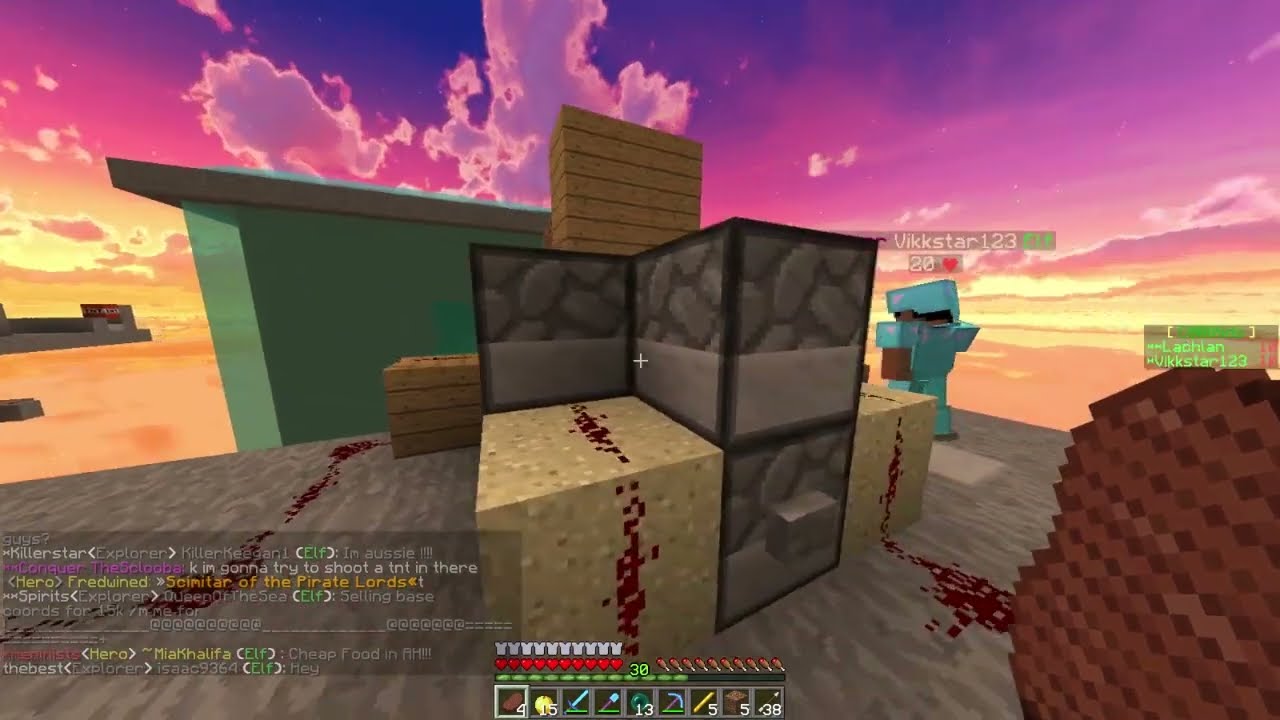The image depicts a pixelated screenshot from an old-school video game, likely from the 1980s or 1990s, shown from a first-person perspective. The focus is on a room with a blue, tiled floor. At the center just right of it, there's a hole or storage space containing bright yellow blocks, possibly bricks of gold, surrounded by brownish objects. The bottom left features a chat area with various messages in white, green, and pink fonts, where users like Permafrost, Champion, Flamehead321, Smeltybrothers, and others are communicating. The messages include phrases like "yes, but you don't have the rank," "OMG, the spam," and "VIK FTW." At the bottom center, there's a user interface displaying a health bar, an energy bar, and multiple weapon icons. Numbers such as 6, 15, 5, and 38 accompany these icons, suggesting various stats or resources. Scattered user names like Lacklan and BKKSTAR123 are seen in the middle right side, indicating an active multiplayer environment.